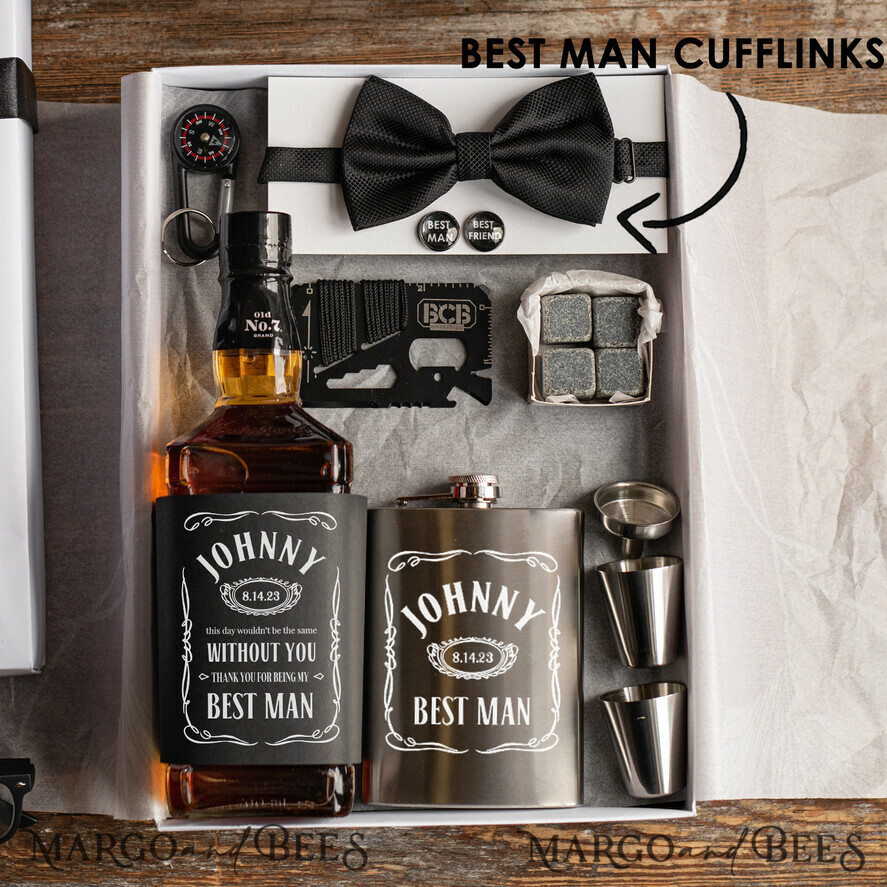The image showcases a detailed wedding-themed gift set, thoughtfully curated for a Best Man. At its center is a bottle of whiskey resembling a Jack Daniels bottle but personalized with the name "Johnny" and the message: "Without you, this day wouldn't have been the same. Thank you for being my best man. 8-14-23." Accompanying the bottle is a silver flask engraved with similar details — "Johnny, Best Man, 8-14-23."

The gift set is neatly arranged within a square box lined with tissue paper. In the top right, there is a black bow tie, and next to it are silver cufflinks labeled "Best Man" and "Best Friend," with an additional emblem marked "BCB." Near the top left lies a small keychain that appears to function as a compass. 

Also included are practical accessories such as two silver shot glasses, a funnel for pouring whiskey into the flask, and a set of four gray items that look like pool table chalk. The lid of the box, adorned with a black ribbon, is visible off to the side.

The box also prominently features labels reading "Best Man Cufflinks, Margo and Bees," reiterating the theme of the gift set. Spectacles can be seen off to the side of the frame, hinting that someone has just admired this elaborate and heartfelt gift.